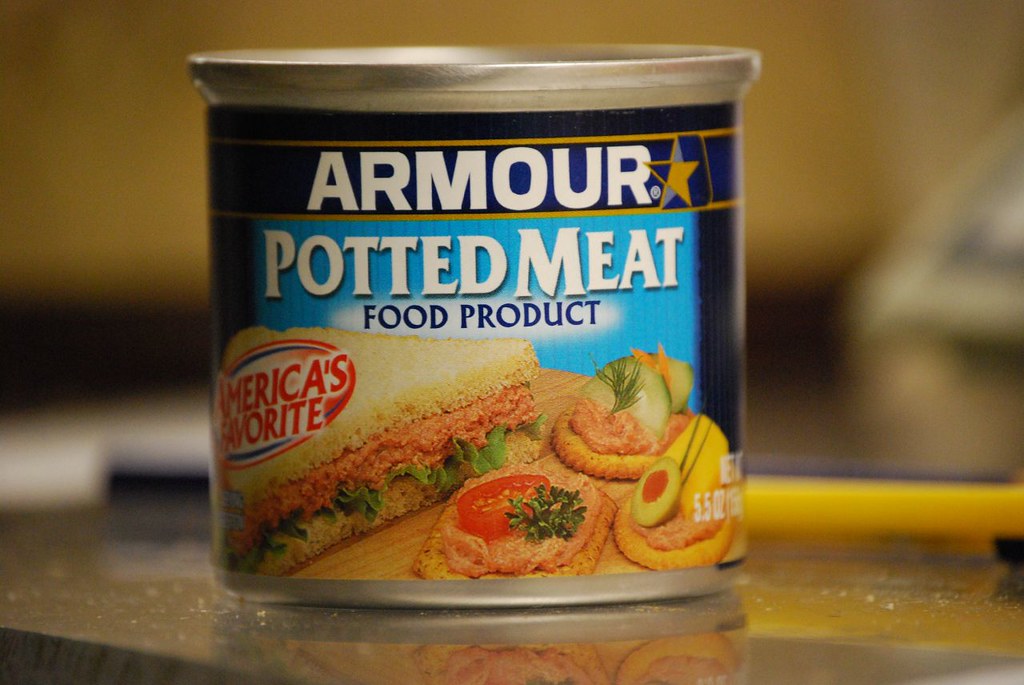This photograph showcases a vintage-inspired, yet possibly contemporary can of food that might be an American or international brand. The label prominently features the word "Armour," spelled in the British style with a "U" (A-R-M-O-U-R), set against a dark blue background highlighted by a golden star on the right. The label is bordered by golden bands at the top and bottom, accentuating its classic appeal.

The center of the can displays a light blue background with the words "Potted Meat Food Product" in bold letters. To the left, the phrase "America's Favorite" suggests its American market presence, contradicting the unusual spelling of "Armour." A detailed illustration of a sandwich graces the label, visually demonstrating its potential use. The sandwich appears to be filled with a soft, spreadable meat product, topped with various vegetables, and nestled between slices of bread. This image aims to highlight the versatility of the potted meat as a sandwich filling or spread, appealing to those looking for convenient meal options.